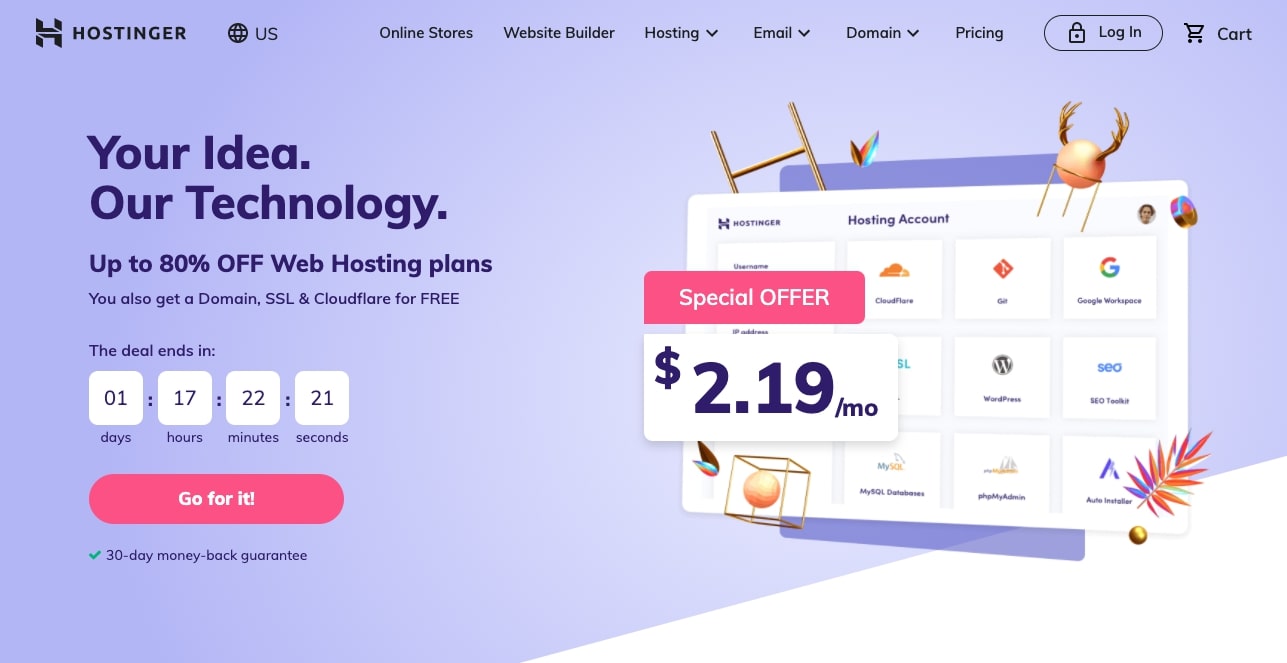The image showcases the landing page of Hostinger's website. Prominently featured at the top is a bold, three-dimensional letter "H," which is stylized to appear as if it is composed of two separate shapes: a "U" and an inverted "U," forming the uppercase "H" when viewed together. The headline of the page reads, "Your Idea, Our Technology," followed by an enticing offer: "Up to 80% off web hosting plans," with a countdown timer indicating the deal ends in 1 day, 17 hours, 22 minutes, and 21 seconds. The special offer price is prominently displayed as $2.19 per month. The page is clearly targeting a U.S. audience and features a visual representation of the hosting account setup. Included in the setup are icons for various services and tools such as Cloudflare, Google Workspace, and WordPress, organized in a grid of 12 blocks arranged in 4 rows and 3 columns.